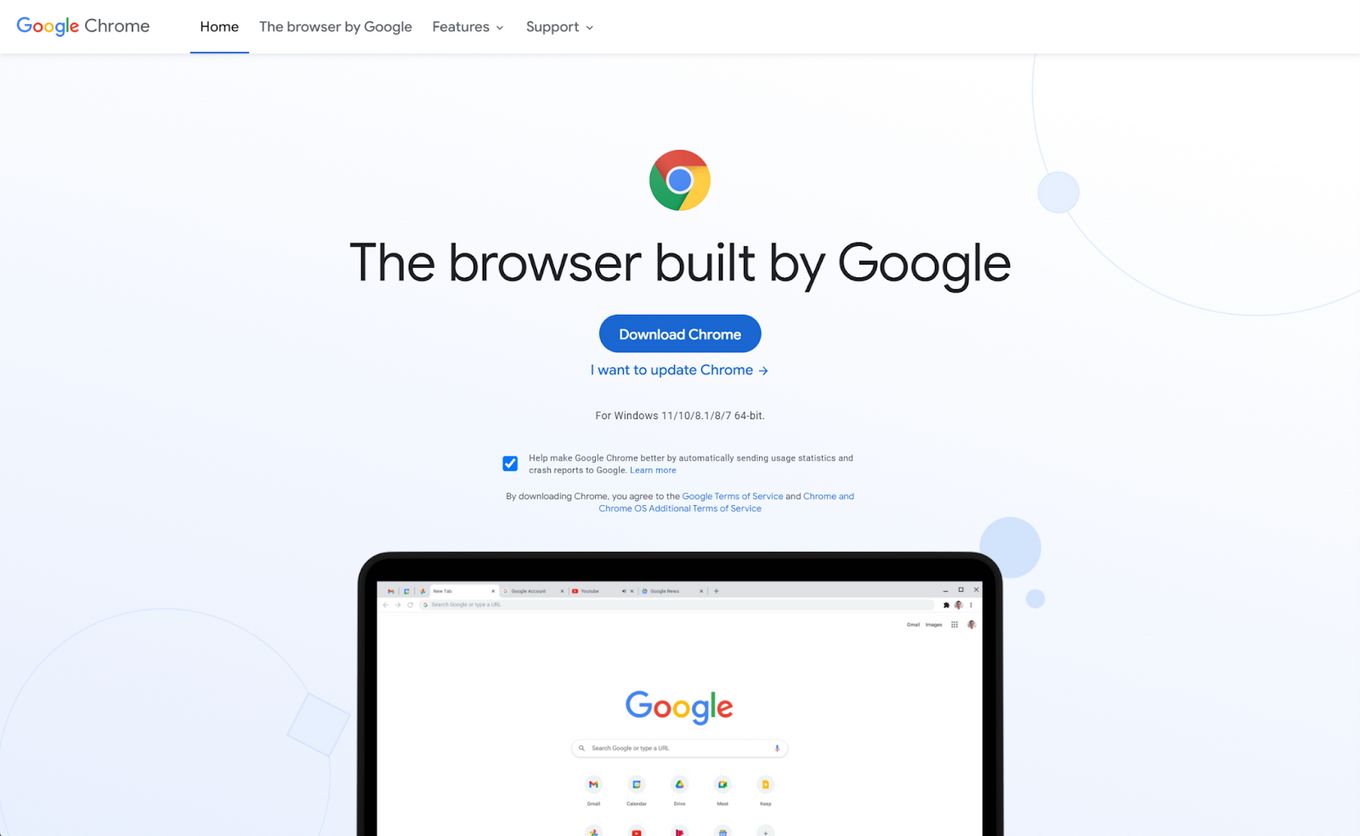The image displays a desktop screen showcasing the Google Chrome homepage, which appears after a user searches for Google Chrome. At the top of the page, there is a navigation bar with links to various sections: "Home," "The Browser By Google," "Features," and "Support." The "Home" section is currently selected, indicated by a blue underline. 

Centrally positioned is the iconic Google logo accompanied by the tagline "The browser built by Google." Below this, a prominent blue button invites users to download Google Chrome. There is also an alternative option for users who already have Chrome but need to update it, marked by a link saying "I want to update Chrome."

Further down, there are specifications for different operating systems, most notably for Windows, though the smaller text details are not clearly readable. Next to these specifications is a blue checkbox, likely indicating a warning or important notice.

The lower section of the image partially shows the top half of an iPad, which is displaying the Google homepage. The iPad screen features the Google logo with a search icon, and below that, ten shortcut icons representing frequently visited sites. The layout suggests that the iPad is superimposed onto the ad, blending technology themes to highlight Chrome’s cross-platform usability.